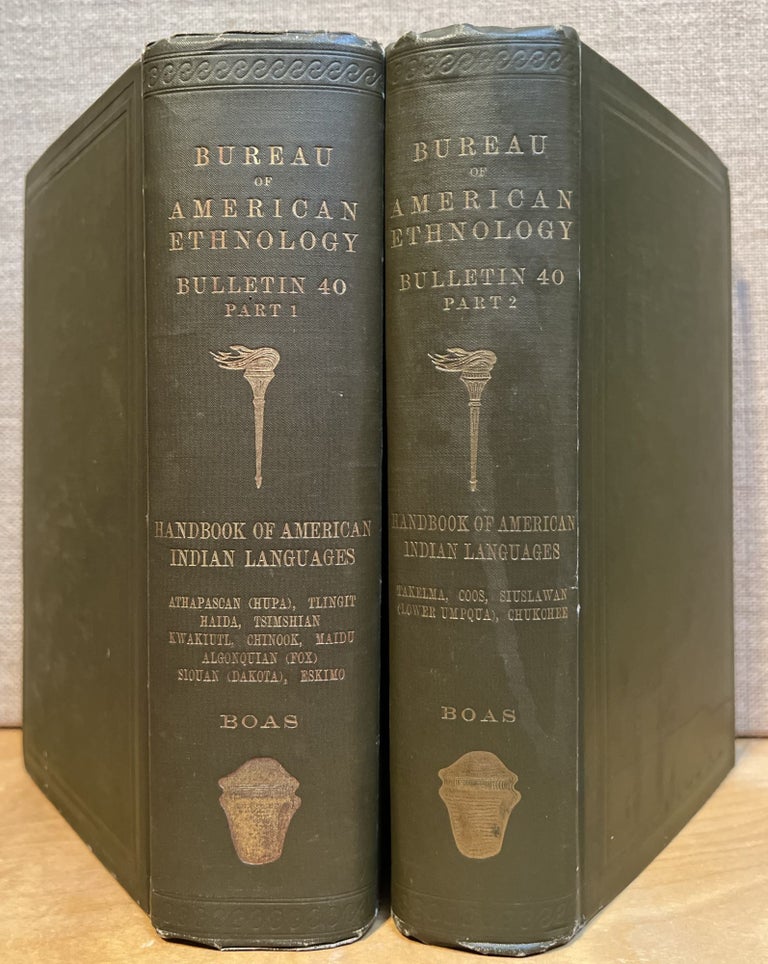This photograph captures two hardcover books placed side-by-side against a tan background, potentially on a light pine surface. The books, bound in dark gray-green leather or canvas, are both from the Bureau of American Ethnology and are titled "Bureau of American Ethnology Bulletin 40." The volume on the left is labeled Part 1, while the one on the right is labeled Part 2. Each spine features a gray, embossed lettering with the subtitle "Handbook of American Indian Languages." Beneath the title, both volumes display an image of a torch, suggesting a publishing house logo, possibly Scribner. Below the torch, there's a list of various indigenous languages covered in the books, which includes Athapaskan, Hupa, Tlingit, Haida, Tsimshian, Kwakiutl, Chinook, Maidu, Algonquin, Fox, Shoshone, Dakota, and Eskimo. The name “Boas” is also noted, possibly indicating an association with Franz Boas. The spines of the books each have a design at the bottom, which resembles a stone grinding implement.